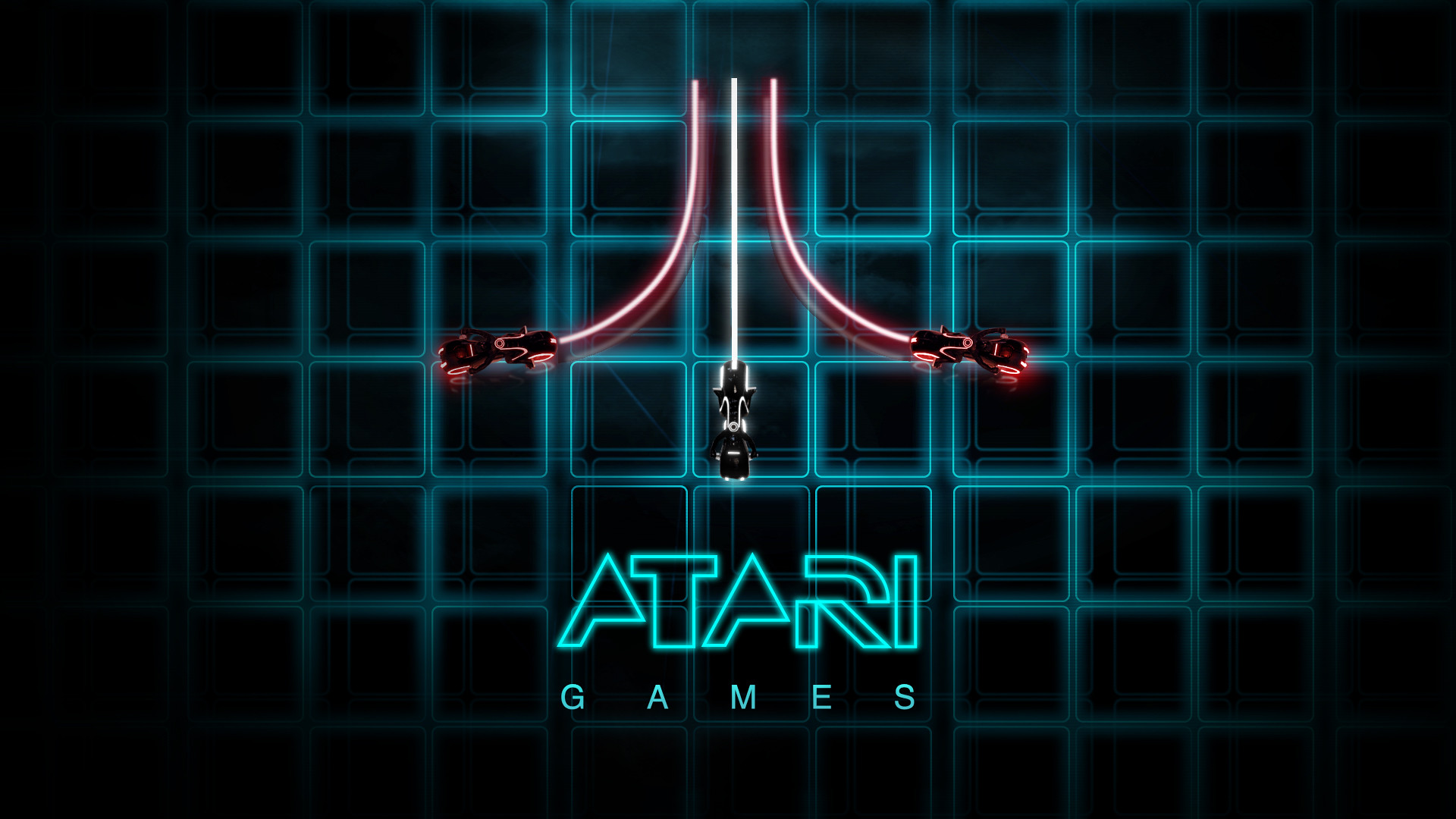This rectangular graphic is evocative of a retro computer game startup screen. The image is dominated by a dark, perhaps very dark blue or black background. Superimposed on this background is an intricate 3D grid rendered in a neon blue, creating a sense of depth and retro-futuristic design. 

At the center of the image, two curved, pinkish-red lines flank a central white line, all depicted with a glowing neon effect, suggesting kinetic energy and motion. These lines are reminiscent of stylized vehicle trails moving in opposite directions, possibly indicating the dynamic spirit of classic Atari games.

Beneath these glowing lines, the word "Atari" is emblazoned in light blue stylized letters that also mimic a neon glow, further reinforcing the vintage aesthetic. Directly below "Atari," the word "Games" is written in a similar light blue, completing the iconic logo. The entire image, with its striking neon elements and grid background, captures the essence of classic Atari branding from a bygone era.